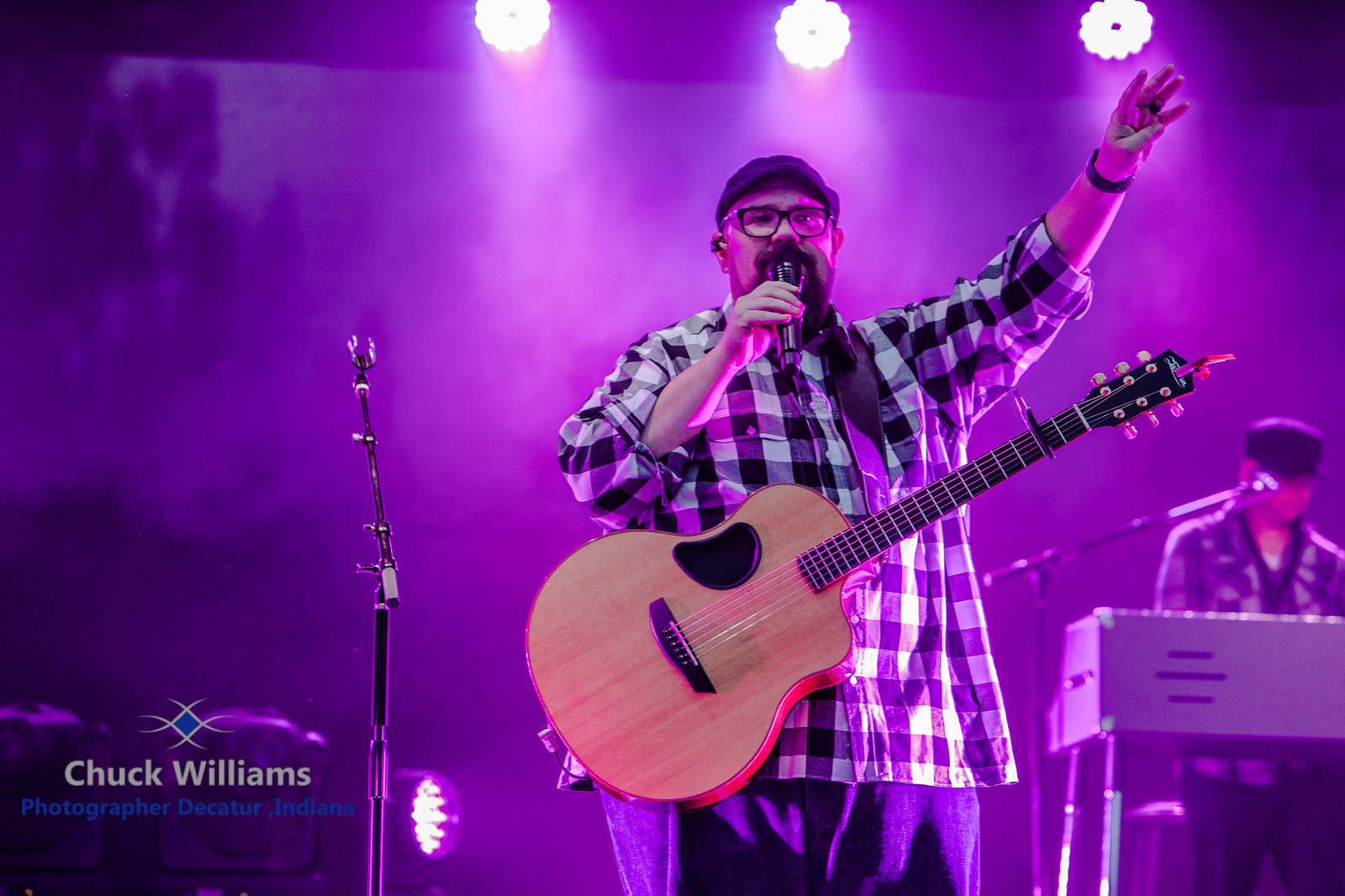In this detailed indoor stage setting, an overweight man stands front and center, passionately performing in a dimly lit, purple-hued room. He wears a plaid shirt, black framed glasses, and a cap, and holds a microphone in his right hand while his left hand is raised. A guitar hangs from a strap across his body. To his right, a keyboardist, head bowed, focuses intently on his instrument with a microphone stand nearby. To the left of the singer, a microphone stand without the microphone stands next to a light. The top of the image features overhead lighting, casting a purple glow throughout the scene. In the bottom left corner, a watermark reads, "Chuck Williams Photographer, Decatur, Indiana," identifying the image's ownership. This compelling image captures the essence of a live music concert.